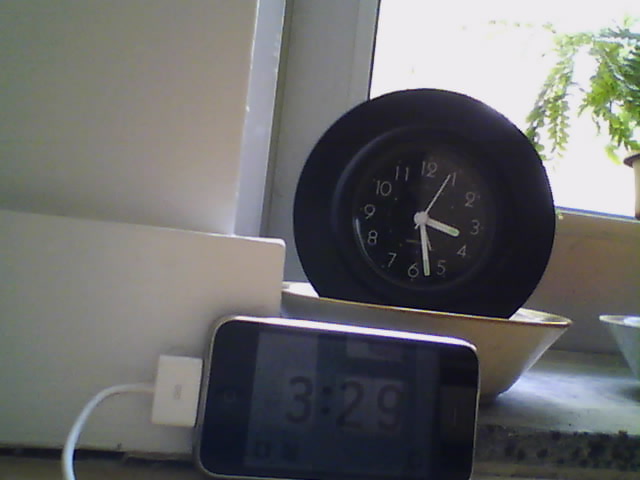In this photograph, a clock is positioned inside a bowl on a table, set against a window backdrop. The analog clock displays the time as 3:27. Natural light filters through the window, suggesting it is late afternoon. In front of the bowl, an iPhone rests on its side, connected to a white charging cable. The phone's screen shows the time as 3:29. A whiteboard is placed behind the phone, possibly to prop it up for the photograph. Through the window, an exterior greenery, likely a fern plant, is visible, adding a touch of nature to the scene.